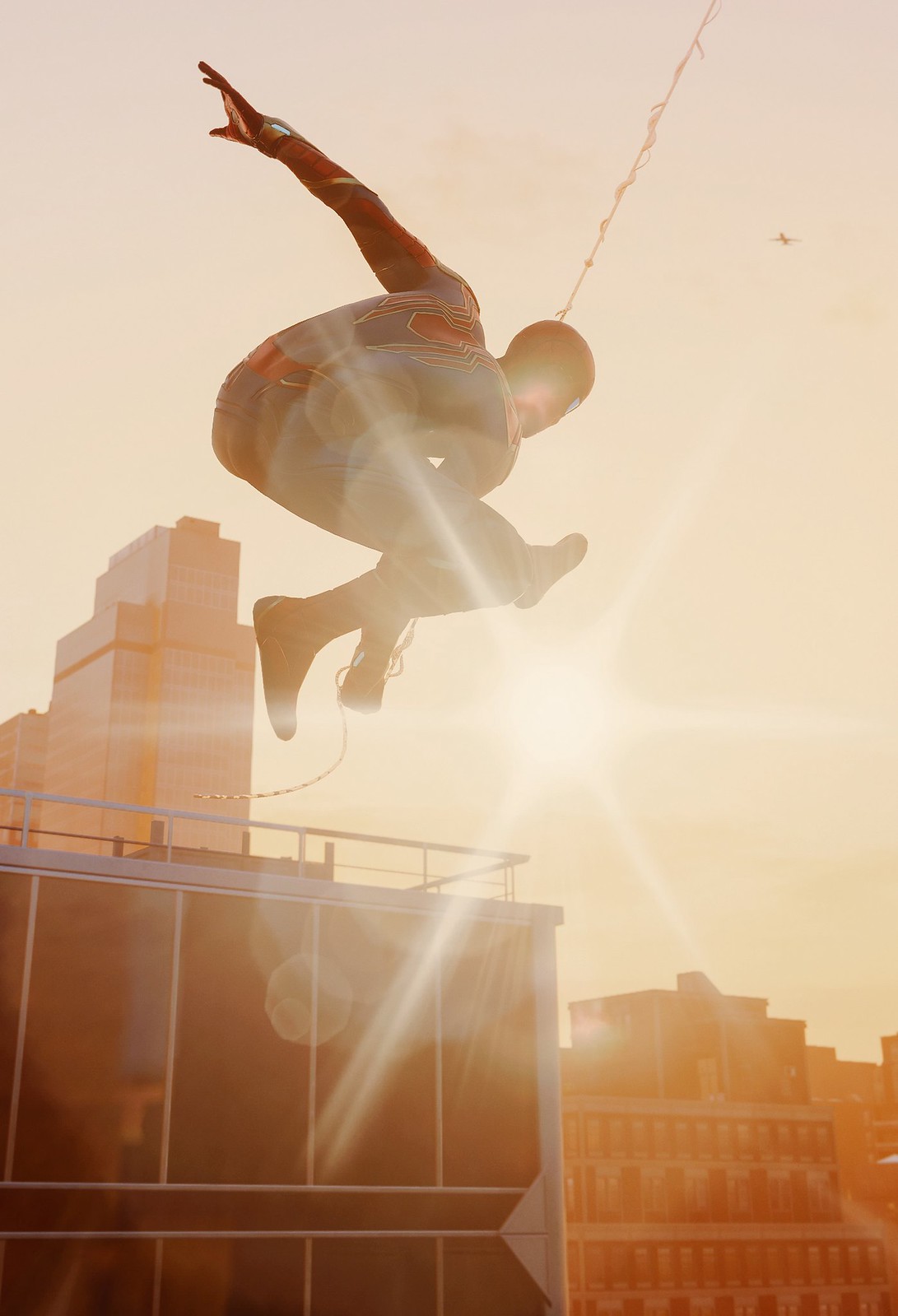In this captivating image from a Spider-Man movie, Spider-Man is captured mid-air, swinging on a web with the cityscape as his backdrop. The scene is set during a late evening with the bright sun casting long, thin rays, producing a stunning orangey hue that permeates the surroundings. The sun's glare in the center adds a dramatic effect, slightly obscuring parts of the image and emphasizing the sunset's vivid colors. Spider-Man is easily recognizable in his signature costume, featuring a red mask, red and blue suit with a prominent red spider emblem on the back, and red, blue, and black shoes. His left arm is bent back at the elbow with fingers stretched out, and his right arm is holding the web. He appears to be in the middle of a leap, with his left leg extended and right leg bent. In the background, tall buildings frame the scene, with a particularly distinctive glass-paneled building near Spider-Man. An airplane is visible in the upper right corner of the sky, adding to the urban atmosphere. The combination of Spider-Man’s dynamic pose and the glowing evening light renders a captivating moment filled with both action and beauty.